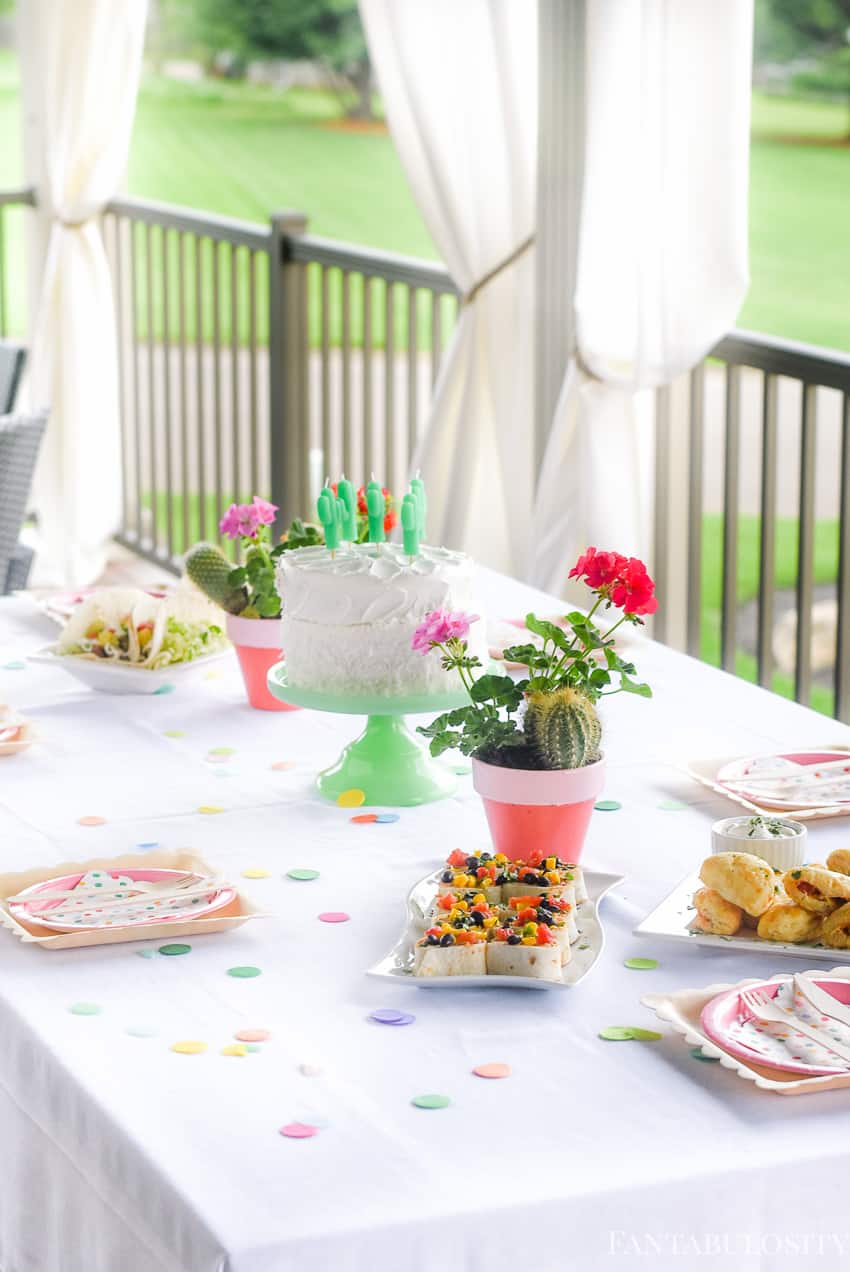This image captures a delightful birthday party scene set on an elegant outdoor porch adorned with white curtains tied to the side, offering a view of a lush green lawn and trees. At the forefront is a pristine table draped in a white tablecloth, sprinkled with pastel pink, blue, and purple confetti, creating a festive atmosphere. The centerpiece is a white frosted birthday cake placed on a light green cake stand, adorned with four charming cactus-shaped candles. Surrounding the cake are various decorations, including small pink plant pots with vibrant pink, purple, and green flowers, some featuring blooming cacti. To the left of the cake are appetizing tacos, while the far right showcases an assortment of hors d'oeuvres, including biscuits and possibly corn and black bean roll-ups. Additionally, the table is set with paper plates in shades of pink and polka dot napkins in coordinating colors, enhancing the celebration's lively and coordinated aesthetic.